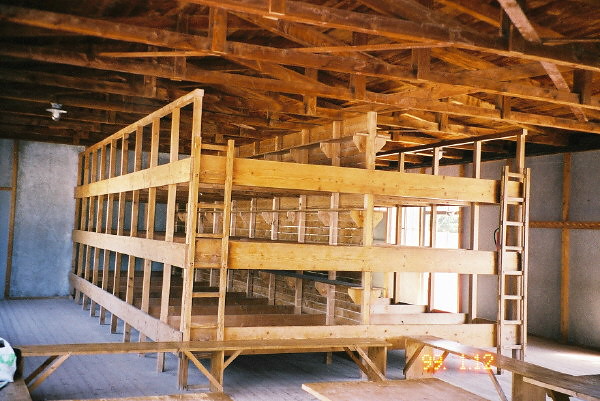The photograph portrays the interior of an unfinished building with white to gray plaster walls and a ceiling comprised of wood panels arranged both horizontally and diagonally to form a triangular shape. The gray floor is made of wooden planks. At the center of the room stands a large wooden structure consisting of three tiers of bunks, made out of light brown boards arranged in parallel rows. Each tier is accessible via identical thin ladders on either side, each ladder featuring seven steps. Additionally, wooden slats run through the middle of these bunks. The rafters above are constructed from reddish-orangish-brown wooden beams. In the foreground, two wooden benches are positioned perpendicularly to the bunk structure. Notably, in the bottom right corner of the image, the numbers "99.1.12" in orange indicate a date.